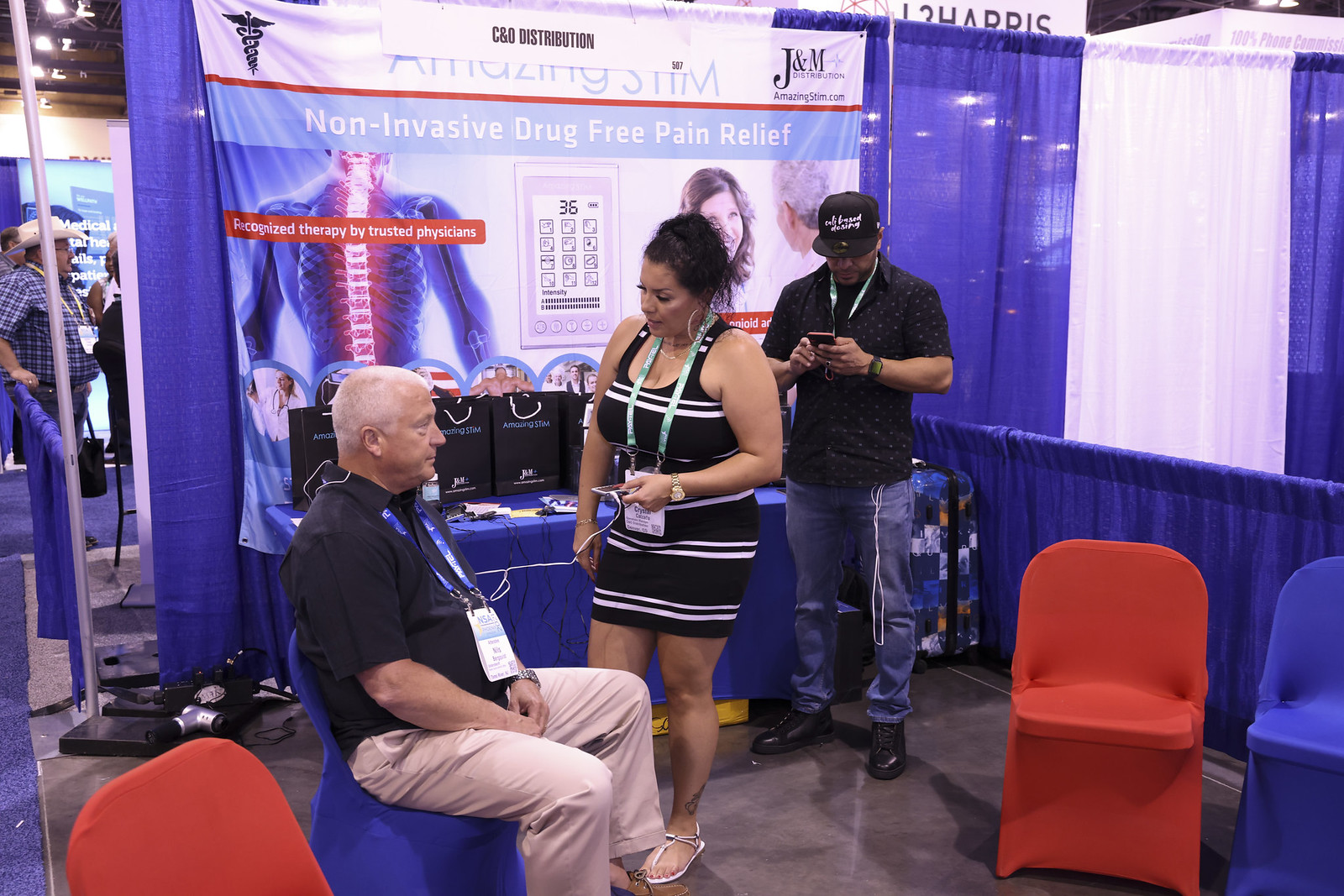In the photo from a trade show or convention, the booth of C&O Distribution features a prominent tarpaulin backdrop with a graphic of a lit-up spine and the text "Amazing Stem - Non-Invasive Drug-Free Pain Relief, Recognized Therapy by Trusted Physicians." A table in the booth, covered with a blue tablecloth, displays pens and branded gift bags.

At the forefront, an older gentleman dressed in a dark blue collared short-sleeved shirt, khaki pants, and top-sider shoes sits in a blue chair. He wears a blue lanyard displaying his ID. Engaged in conversation with him is a woman wearing a black and white tank top dress and white sandals, with a green lanyard around her neck. Her smartphone is connected to a monitor, presumably demonstrating the therapy. Behind her, a man in jeans, a black collared shirt with gold circles, a black baseball hat, and a green lanyard, stands absorbed in his smartphone. The scene captures a moment of interaction and interest in the non-invasive pain relief products being showcased.